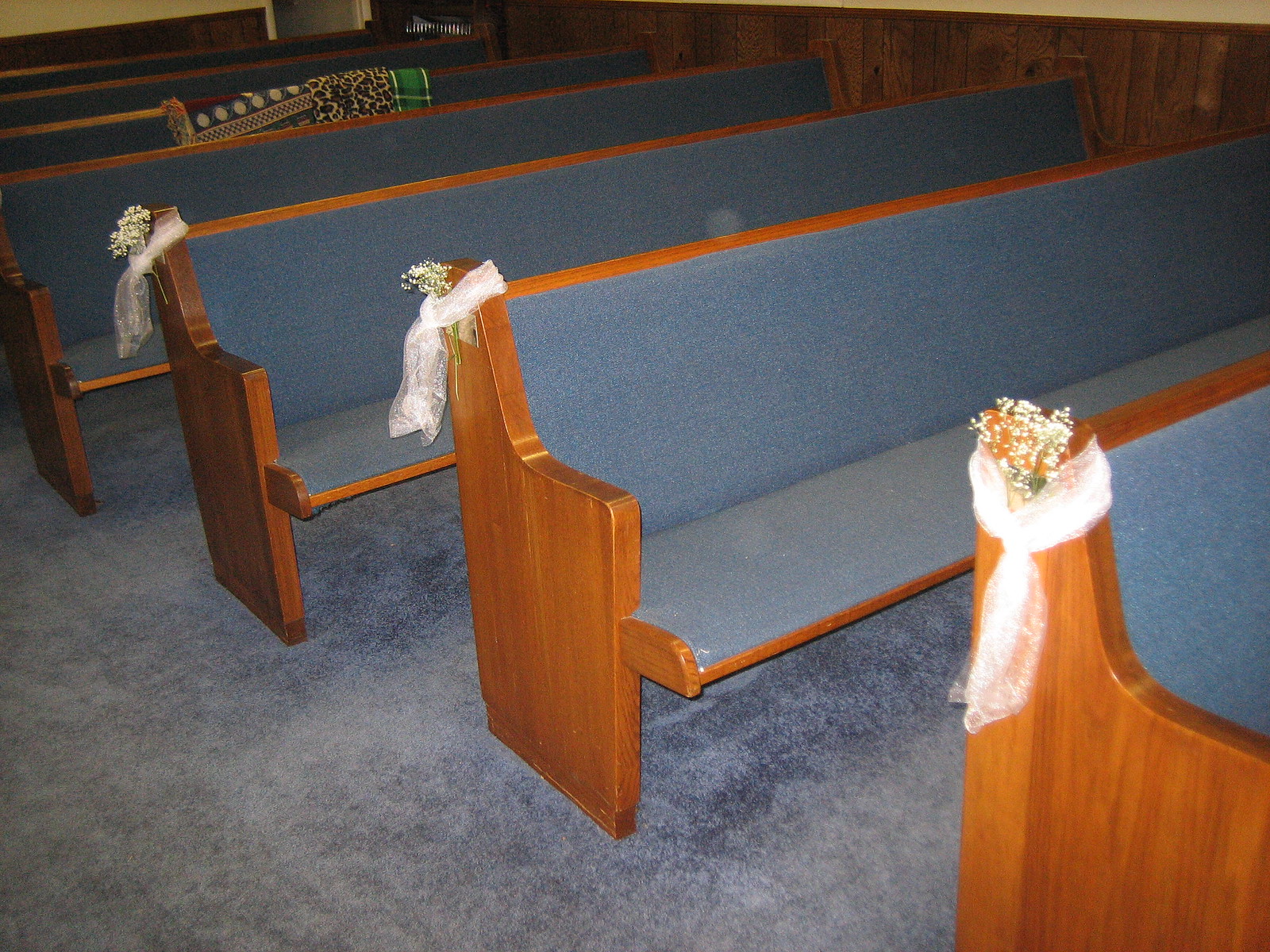This photograph captures an interior view of what appears to be a church, decorated for a wedding. The scene features seven rows of long, wooden pew benches, each fitted with matching blue cushions on the seats and backrests. The flooring is adorned with blue carpet, complementing the cushioned pews. The ends of the benches are adorned with delicate wedding decorations: white lace fabric tied around the top edges, accompanied by petite bouquets of baby's breath flowers. Notably, in one of the back rows, two blankets—a green plaid one and a leopard print one—are draped over the pew, adding a personal touch to the setting. The walls of the room are wooden-paneled, completing the serene and warm ambiance of the space.